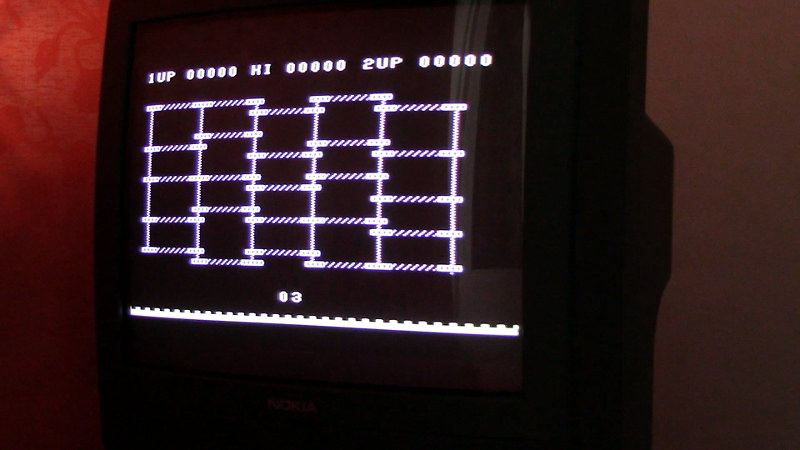This photograph depicts a vintage arcade game displayed in a dark indoor setting. The arcade machine, which is predominantly black, features a large, square screen with slightly pixelated graphics showcasing a classic game. The game screen is dominated by a mesh of vertical lines intersected by horizontal bars, creating a ladder-like pattern. At the top of the screen, there's familiar arcade game text such as "1UP" and "2UP," indicating player statuses, along with the high score display. Above the lines on the screen, there's a white number three. The bottom of the screen displays a white horizontal line adorned with black dots, forming a distinct pattern. The background of the photograph has a vibrant red hue which appears brightest towards the top right due to the light source, gradually fading into darker shades and almost black as it moves downwards. Hints of a dark purplish-gray shade are also visible on the right-hand side of the image, adding to the moody atmosphere.